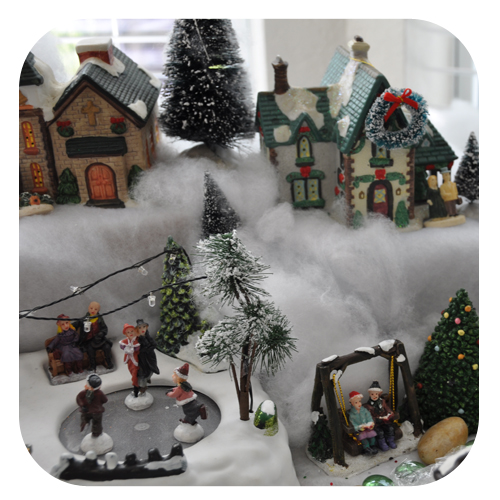This detailed indoor scene captures a festive Christmas display meticulously set up on a table. The backdrop features a white-trimmed window against a gray wall, illuminated by the soft ambient light. In the foreground, cotton material is artfully spread out to simulate a snowy landscape. The display is arranged in two horizontal rows: the upper row showcases a charming Christmas village with an assortment of decorated houses, including a white two-story house with a green roof and another two-story house with brown walls and a green roof. Each house is festively adorned with wreaths and colorful Christmas decorations, and one house features a church with a cross on its summit and a striking gold door, symbolizing the essence of Christmas.

Scattered among the houses, a variety of festively adorned trees, miniature pine cones, and tiny figurines bring the village to life. The figurines include people in holiday attire ice skating on a rink beneath a sprinkle of snow, while others watch from a nearby bench. In addition, there's a swing set where people sit, enjoying the seasonal atmosphere. The lower row complements the scene with more holiday figures, including skaters gliding across the "ice" and trees dressed in festive lights, creating a picturesque and heartwarming Christmas tableau.